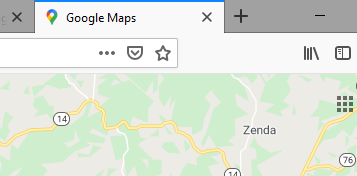This is a colorful screenshot of a Google Maps webpage. The top of the image prominently displays the Google Maps tab, complete with the iconic multicolored location pin. Although the bottom portion of the image is cut off, a segment of the map is still visible. A meandering yellow line, representing a route, arcs from the left edge of the image, dips toward the bottom and then rises again. Key markers along this route indicate numbers "14" and "76" towards the bottom right corner. The only discernible text on the map is the location "Zenda," suggesting a point of interest or destination. The image has a wider horizontal span compared to its height.